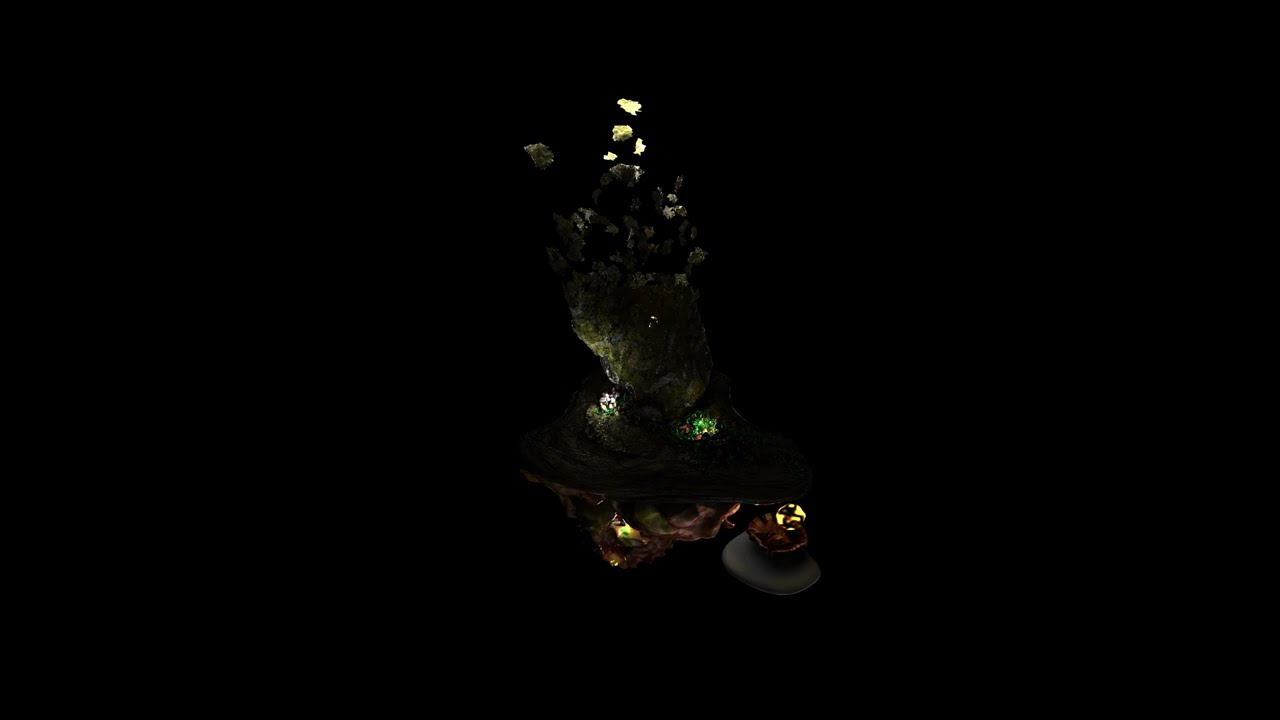The image is dominated by deep blackness, with a horizontal rectangular layout. At its center is an enigmatic, organic-looking sculpture that might be a computer graphic or an illustration. This sculpture, resembling some form of plant or moss, is sporadically illuminated, revealing dark green tones interspersed with white and red flowers. The structure has a complex shape, rising and curving intricately toward the top, where it features more floral elements and possibly stone-like pieces. Below the central figure lies a ledge strewn with rocks and dirt, where a flat gray stone holds a bowl containing a shiny, marble-like object. Despite the scarcity of light, the scattered pools of illumination offer just enough visibility to hint at the mysterious, almost cavernous setting of this scene.